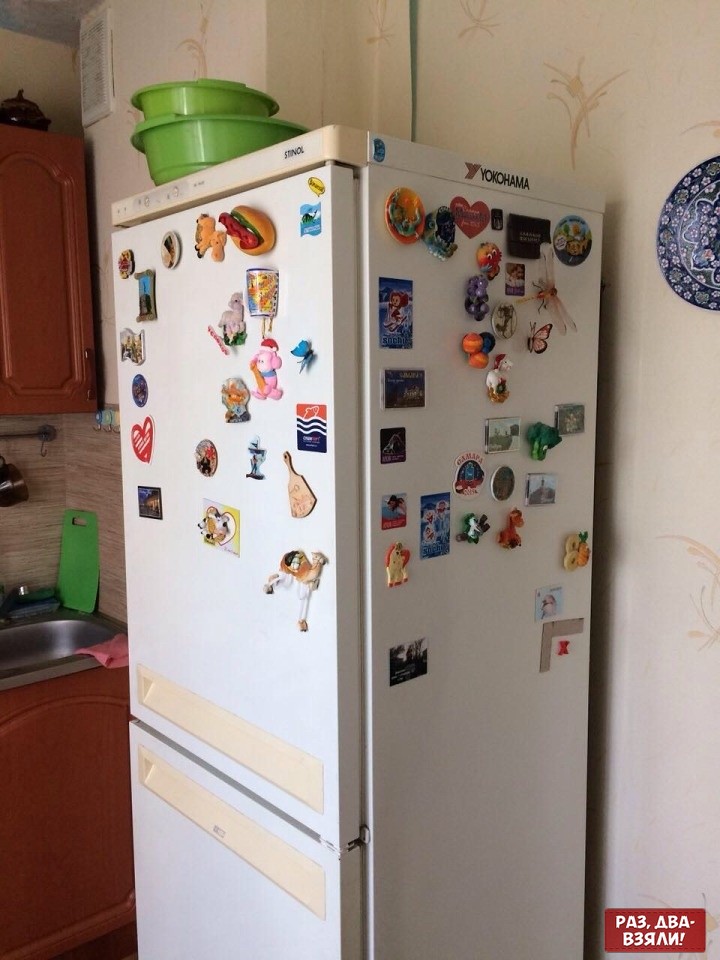This detailed photograph showcases a kitchen with a primary focus on a tall, white refrigerator adorned with a variety of colorful magnets depicting different characters, animals, and memorabilia. The top right corner of the fridge features a magnet that says "Yokohama," while other magnets include images of camels, a hot dog, hearts, and some with Cyrillic writing. Above the fridge, two green bowls are stacked one inside the other. The refrigerator is situated against a pale white wall decorated with a faint pink floral design, complemented by a circular blue plate with white flowers hanging on the upper right side.

To the left of the fridge, there is a section of the kitchen showing brown cabinetry both above and below a stainless steel sink. On the sink, a light green cutting board is leaning in the corner, and a yellow towel can be seen nearby. The wall beside the sink features a gray, tile-like backsplash. Notably, there is a reddish-brown rectangular marking with white writing, which includes the text "PA3.ABA, B3R, upside down, V, N," or similar, located in the bottom right corner of the image. The kitchen evokes a cozy atmosphere with its mix of functional elements and personalized decor.